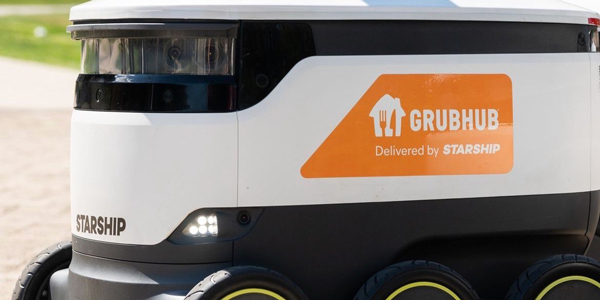This close-up photograph captures a predominantly white delivery drone vehicle named "Starship". The vehicle's design features a prominent white stripe on top, and adjacent to it on the left side is a clear area revealing a device or camera behind glass or plastic. Below this device, a black stripe slopes upward to the right, adding to the drone's sleek appearance. The bulk of the vehicle is covered in plain white cladding, which features black text on the left at the bottom that reads "Starship." Centrally located on this cladding is an orange emblem angled at 45 degrees on the left and extending into a rounded rectangle shape. Inside this emblem is a white logo depicting a house with an orange fork and knife, accompanied by the text "Grubhub" in white letters and "Delivered by Starship" in thinner white text beneath it. 

Underneath the cladding, there is another black section containing lights situated near the "Starship" text. The drone rests on three visible black rubber tires, each adorned with a yellow outline and featuring a black hub. Although fully visible from the side, the top and bottom parts of the vehicle are not shown in the image. The front of the vehicle includes two forward-facing lights and a clear plastic area which might be assumed to allow visibility of the interior mechanisms. The device gives an impression of having owl-like eyes due to the reflections, but this is speculative. The machine's purpose seems clear in the context—serving as a delivery device for Grubhub.